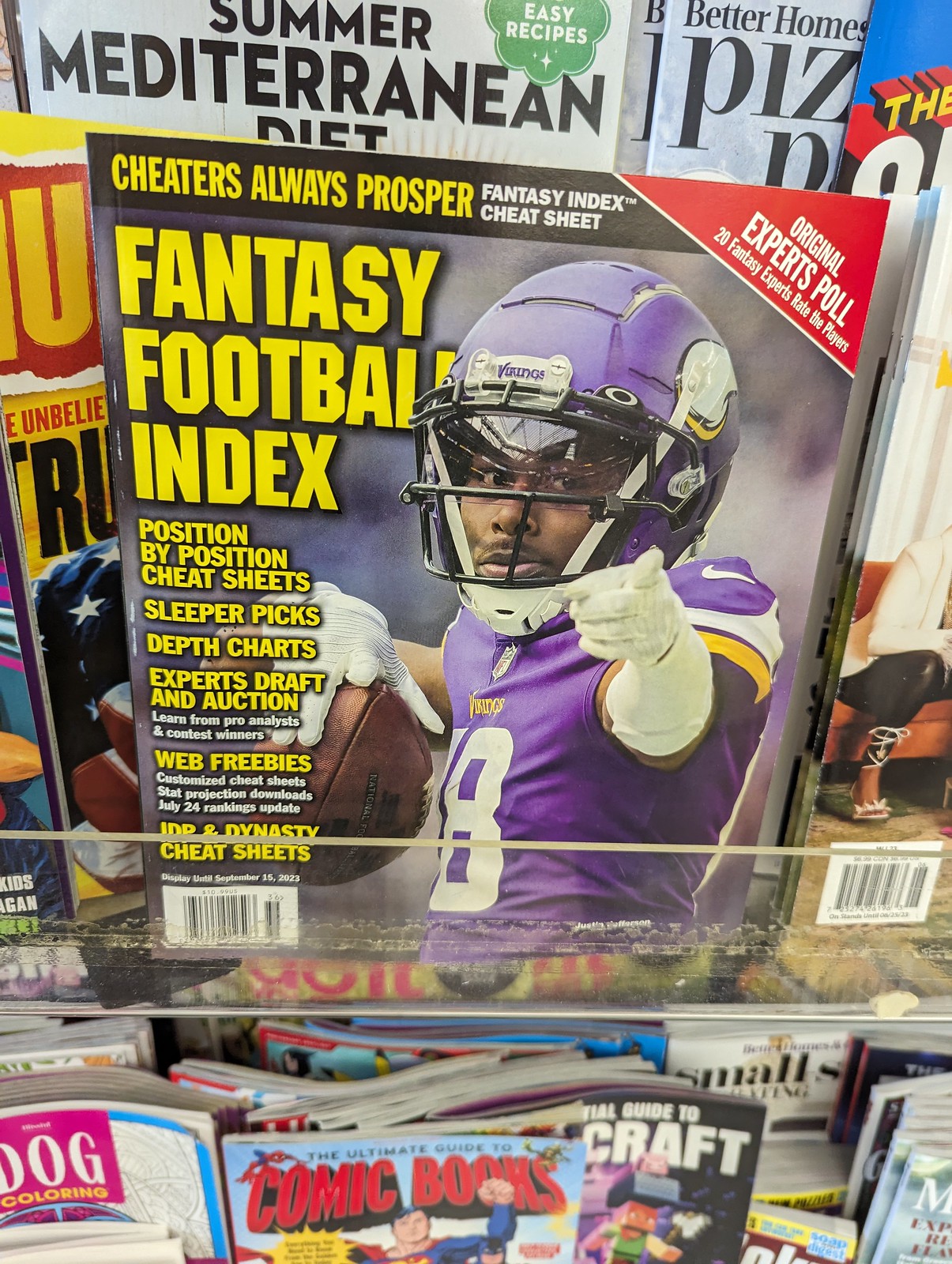This image shows a magazine rack featuring a variety of publications, prominently displaying a Fantasy Football Index magazine at its center. The magazine's cover features a Minnesota Vikings player in full uniform and helmet, pointing and holding a football. Above the player's image, the title "Cheaters Always Prosper Fantasy Index Cheat Sheet" is prominently displayed. A red triangle in the upper right corner announces an "Original Experts Poll: 20 Fantasy Experts Rate the Players." 

Details on the left side of the cover, listed in yellow text under the main title, include "Position by Position Cheat Sheets, Sleeper Picks, Depth Charts, Expert Draft and Auction, Learn from Pro Analysts and Contest Winners." Further information includes "Read Freebies, Customize Cheat Sheets, Stat Projections and Downloads," and "July 24 Ranking Update, IDP and Dynasty Cheat Sheets." 

Other magazines on the stand include a comic book, a dog coloring book, a guide related to Minecraft, a summer Mediterranean diet magazine, and an issue of Better Homes and Gardens. The Fantasy Football Index magazine indicates it should be displayed until September 15th, 2023, signifying its recent release.